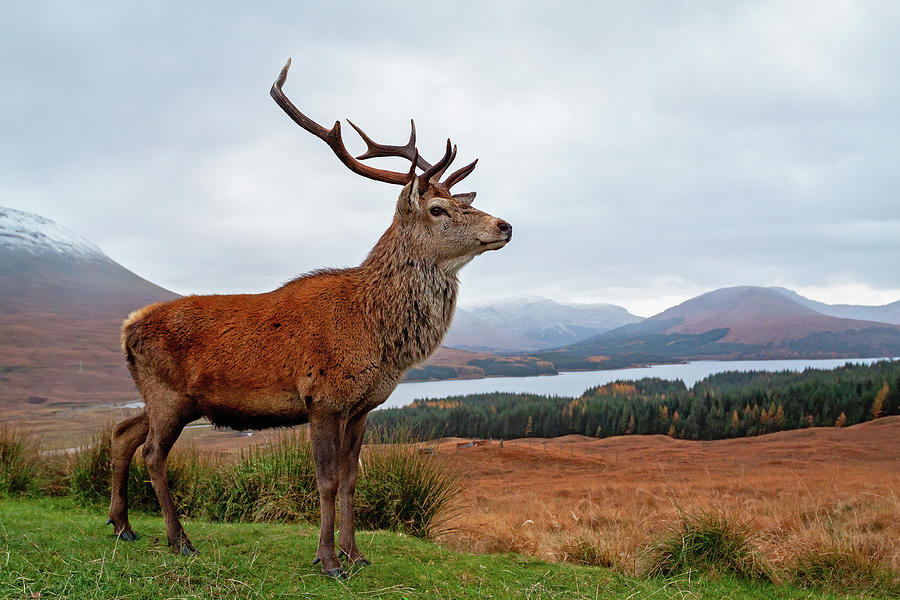This breathtaking, wide-angle color photograph captures the serenity and majesty of pure nature. In the foreground, a magnificent adult elk with a powerful build and large, impressive antlers stands tall on a patch of green grass. The elk, with its rich brown fur that lightens slightly towards the neck, looks directly at the camera, striking a commanding and regal pose. Its back left leg is subtly pushed backward, adding a natural grace to its stance.

The background unfolds into a sweeping tableau of diverse natural elements: a stretch of brown grass transitions into a mix of dense green pine trees and brush. Beyond this, a tranquil lake mirrors the rugged majesty of distant mountains, and the entire scene is crowned by a sky thick with clouds. The image is devoid of any human presence, allowing the viewer to fully appreciate the untouched wilderness. Overall, this photograph is a stunning composition of an elk in its natural habitat, standing solitary yet powerful amidst the vast and varied landscape.